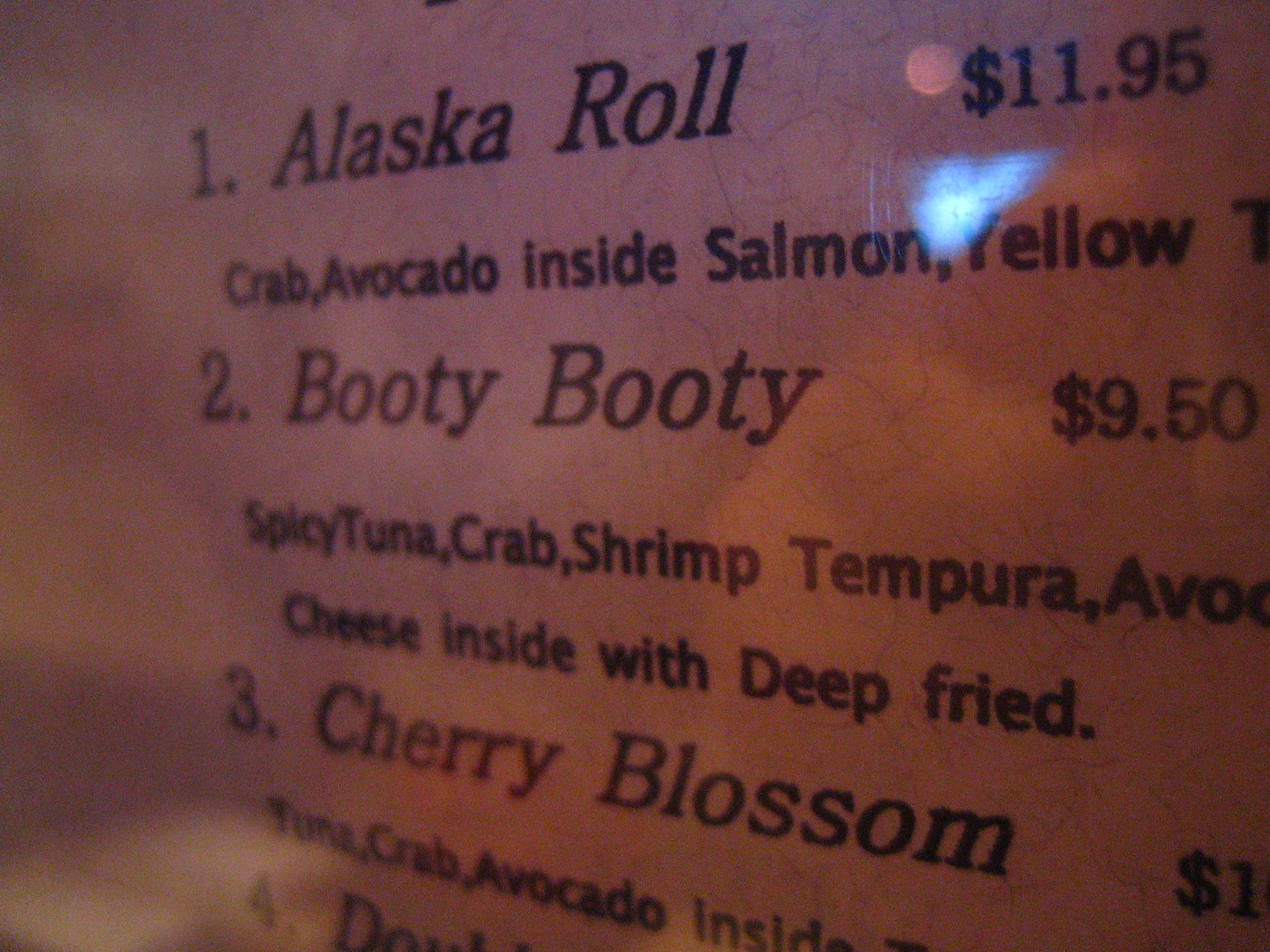This photograph captures a close-up of a restaurant menu predominantly featuring seafood dishes. The menu, which is printed on white paper with black font, is set against a dark background. A reflection from a cell phone's flashlight suggests the picture was taken in a dimly lit environment. 

The first item listed is the Alaska Roll, priced at $11.95. This roll consists of crab and avocado, wrapped inside yellow salmon. The next item is whimsically named Booty Booty, costing $9.50. It contains a combination of spicy tuna, crab, shrimp tempura, avocado, and cheese, all deep-fried, with cheese included inside. 

The third dish, called Cherry Blossom, has its price partially obscured, showing only "$1.00," making it difficult to determine the exact cost. This item includes tuna, crab, and avocado, with additional ingredients cut off in the image. The fourth menu item, which begins with the word "Double," is similarly cut off, making the full name and description unreadable.

This image provides a glimpse into the menu's offerings, though some details remain hidden due to the angle and reflection in the photograph.